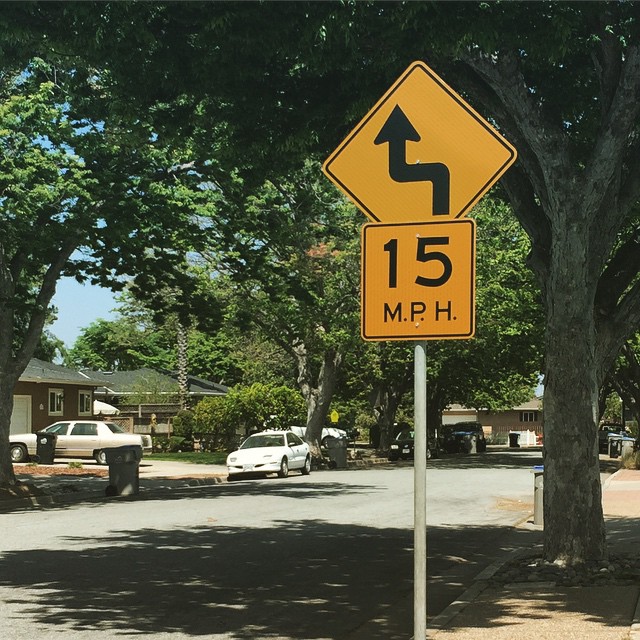This photograph captures a residential neighborhood street on a sunny day with a clear, Carolina blue sky. Prominently featured in the foreground is a silver pole supporting two road signs. The lower sign is a yellow square with black borders, stating "15 MPH," indicating the speed limit. Above it, there is a yellow diamond-shaped sign with a black border, displaying a jagged arrow warning of an upcoming sharp left turn followed by a right; this suggests the street is not a cul-de-sac but has a hidden turn. The street is lined with one-story homes and bungalows, mostly on the left side of the image, interspersed with both tall palm trees and various regular trees casting large shadows. The presence of garbage cans pulled to the curb suggests it is trash day. Numerous cars are parked along the street and in driveways, and a sidewalk runs alongside the road, emphasizing the neighborhood's residential nature.